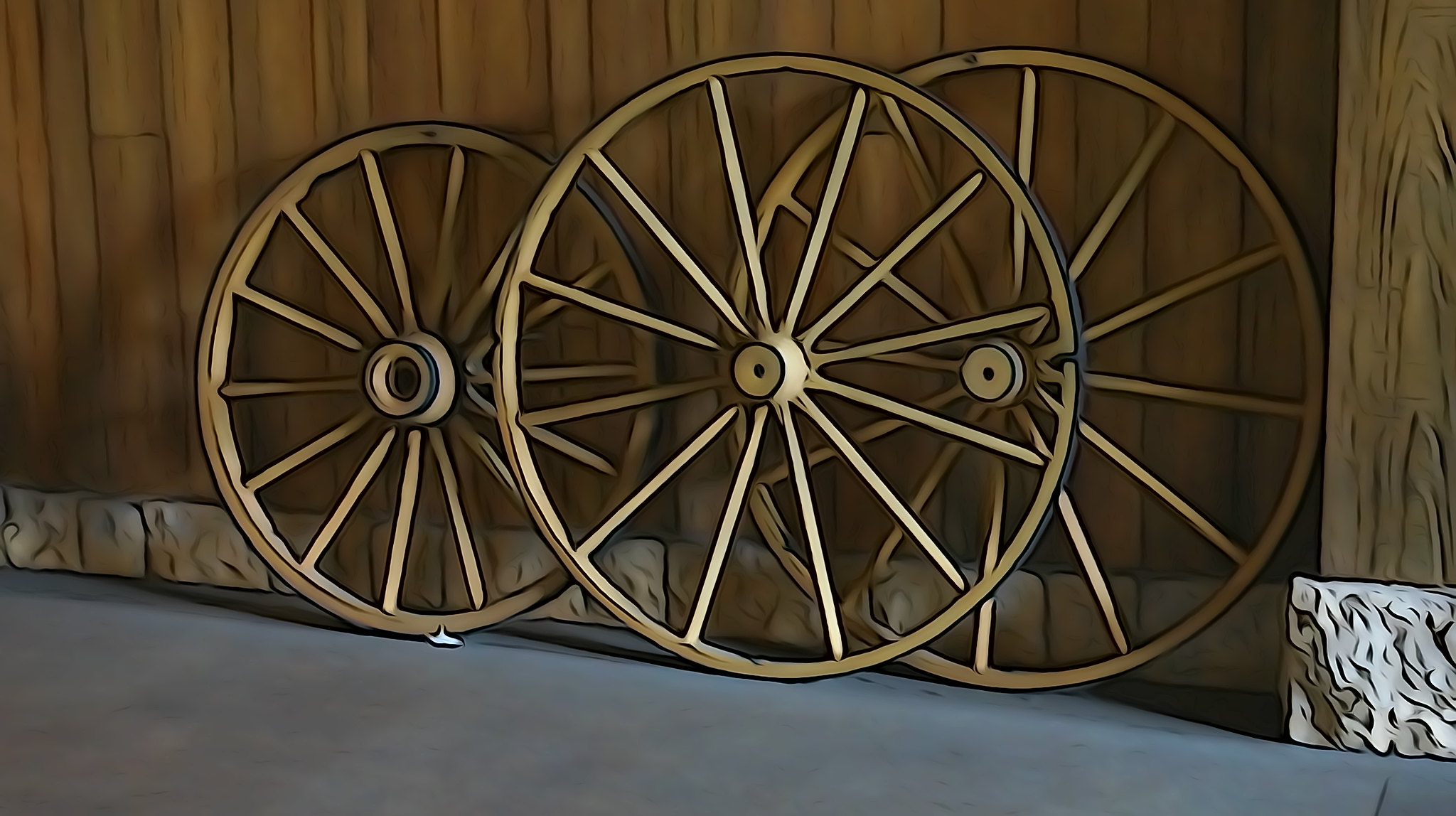This detailed digital artwork, resembling a highly realistic yet cartoon-like style reminiscent of Telltale games, features three wagon wheels leaning against a vertical wood-paneled wall. The scene is accentuated by the thick black outlines typical of cell shading. The wooden wall, composed of vertical planks, is set against a backdrop of rectangular stones lining its base. The bottom foreground displays a gray pavement area, with a small section of textured white rock in the bottom right corner. The three wagon wheels, sporting a slight yellowish hue with black outlines, are arranged with the smallest wheel at the back left, a larger wheel to its immediate right, and another large wheel positioned prominently in the foreground, partially overlapping the other two. This tranquil scene, devoid of people, animals, or flora, captures a serene and static moment in vibrant detail.